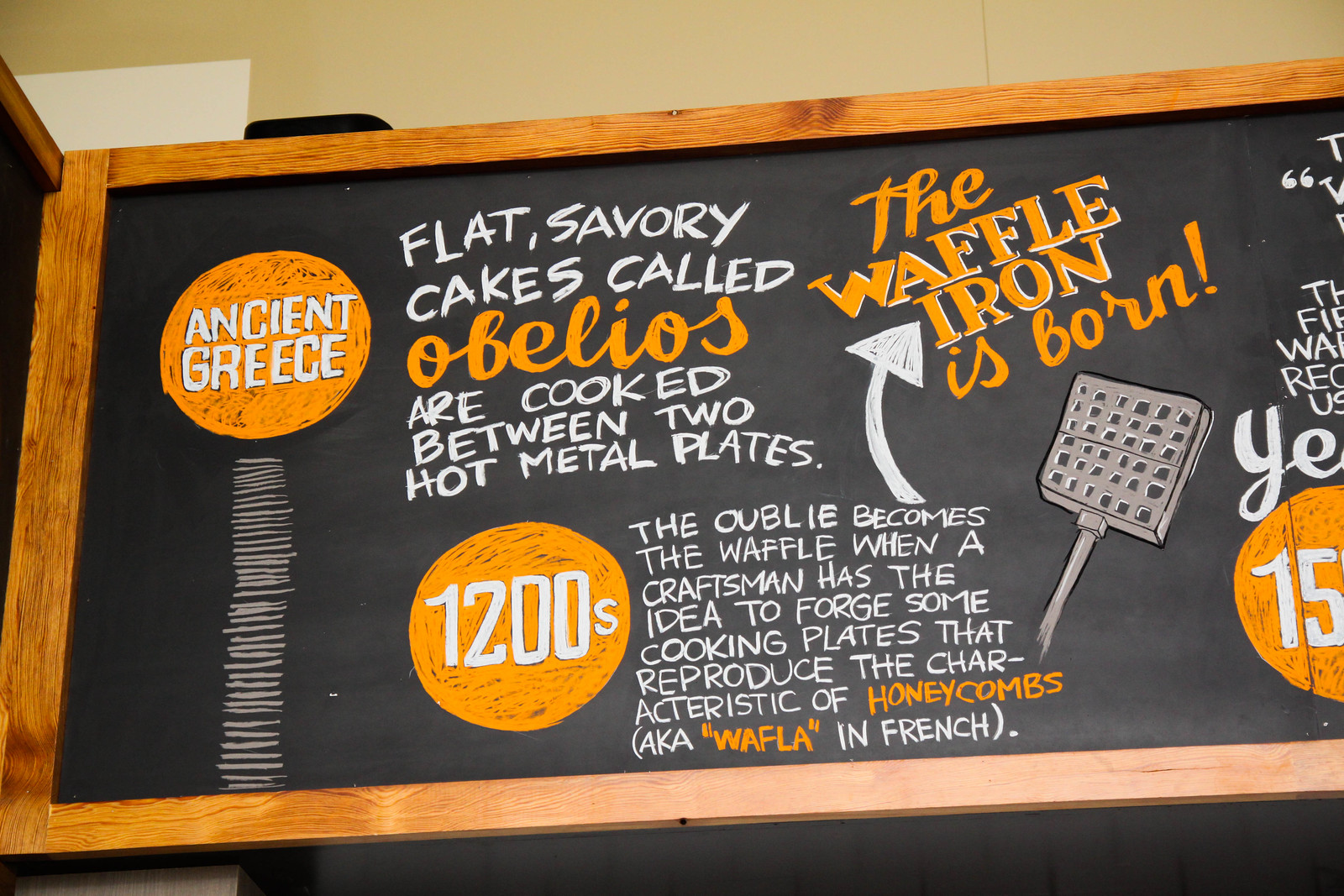This image depicts a chalkboard sign, possibly displayed in a restaurant or museum, framed with medium brown wood. The sign narrates the historical evolution of the waffle. On the left, within an orange circle, are the words "Ancient Greece" written in white letters. Continuing to the right, it details that "flat savory cakes called Obelios were cooked between two hot metal plates" in the 1200s. The text explains how obelios eventually transformed into waffles when a craftsman conceived the idea of forging cooking plates that mimicked the structure of honeycombs – known as "waffler" in French – leading to the birth of the waffle iron. A graphic of a waffle iron is included, suggesting the invention's timeline. The chalkboard features white and orange lettering, adding visual distinction to the historical context provided.